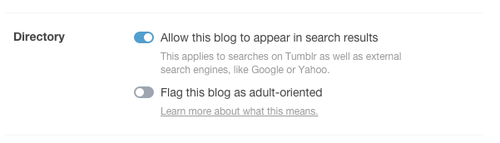In this detailed screenshot, starting at the top, there's a thin, light gray horizontal line stretching from the left to the right. Directly below this, on the left side, appears the word "Directory" in black text. Immediately to its right, there's a small blue oval-shaped button with a white circle on its right side, resembling a check mark. Moving further right, the words "Allow this blog to appear in search results" are displayed. Beneath this statement, in a lighter shade of black or light gray text, it reads, "This applies to searches on Tumblr, as well as external search engines like Google or Yahoo."

Continuing downward, there's another oval-shaped button, this time with a gray color and a white circle on its left side, indicating that the toggle is switched off. Adjacent to this button is the phrase "Flag this blog as adult-oriented." Below this, in the same light gray color, is a sentence with underlined text stating, "Learn more about what this means." Finally, at the very bottom of the image, another thin, light gray horizontal line spans across, marking the page's end.